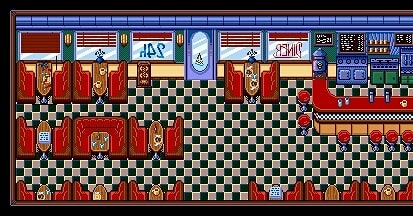This image appears to be a pixelated screenshot from a video game, depicting an indoor scene. The rectangular frame showcases a room designed resembling a dining or seating area. Positioned centrally at the top is a purple-colored door, suggesting an entrance or exit. Flanking the door on the left side are three windows, while the right side features two windows, all contributing to a symmetrical layout. The floor presents a checkered pattern in black and white, enhancing the retro aesthetic. Scattered throughout the room are several brown tables, each accompanied by red chairs. The chairs are neatly arranged on either side of each table, with the red seats adding a pop of color against the subdued tones of the room’s decor.